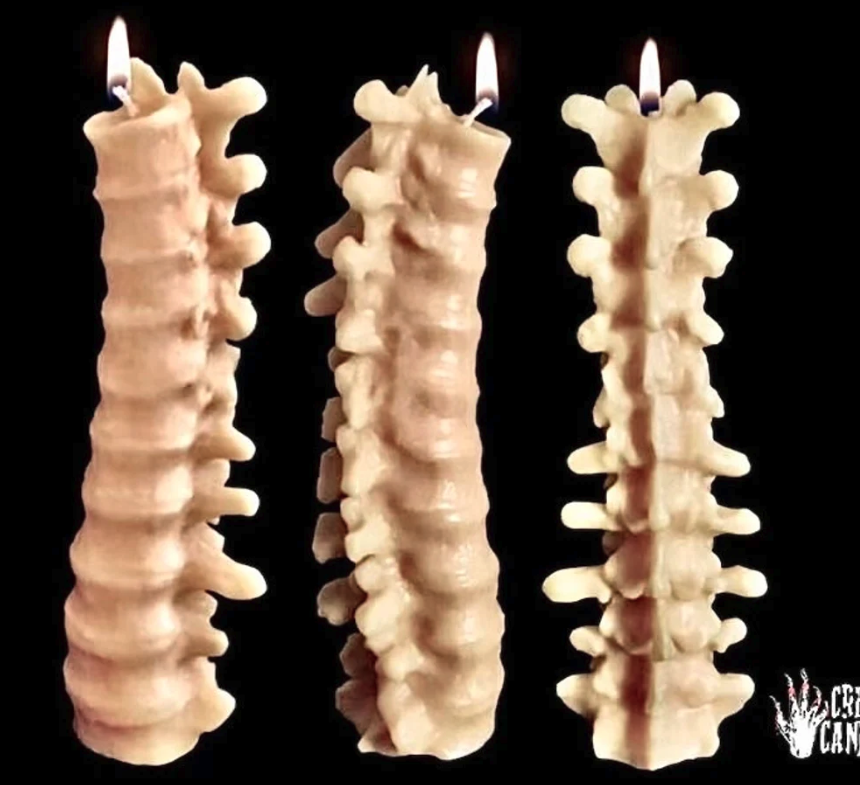In this photograph, a striking composition is set against a black background. Dominating the scene are three lit candles, each meticulously crafted to resemble human vertebrae. Their wax is beige in color, giving them a realistic bone-like appearance. These candles, with flames that flicker gently atop, feature detailed vertebral shapes extending outward, adding to their intricate and somewhat eerie design. Positioned in different orientations, one candle appears inverted and facing the viewer, while the other two seem to be aligned towards each other. At the bottom right corner of the image, there is a partial emblem displaying a hand and some incomplete text, possibly "C-A-N", but the rest is obscured. The photograph highlights the exquisite detail of the candles' vertebral design and the subtle interplay of light against the dark backdrop.